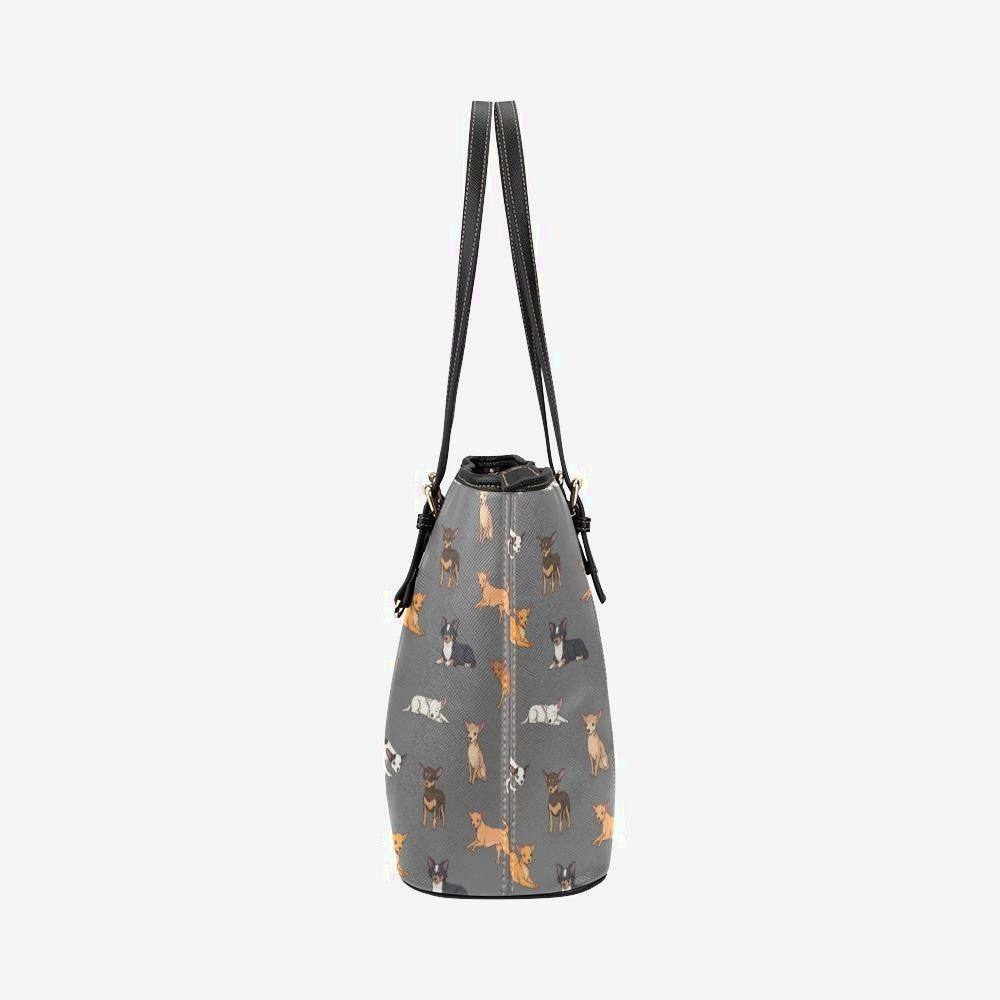This photograph features a narrow, tall handbag made of shiny gray fabric adorned with a repeating pattern of cartoon chihuahuas. The chihuahuas exhibit various poses and colorations, including white, tan, black and white, and reddish-brown hues. The side seam, stitched in white, is visible along the bag's front. Black leather edges frame the bag, and long, slender leather straps stretch upwards, disappearing out of the frame. The straps are attached to the bag with silver buckles. The image is set against a clean, white background, making the handbag appear as though it is floating in mid-air, giving it a professional product photo feel.